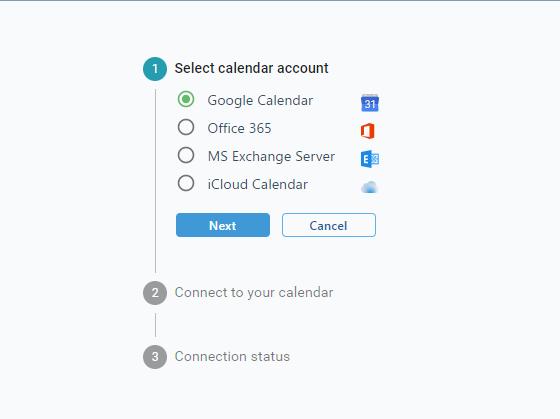The image depicts a screen capture from a computer application with a predominantly gray background. At the very top, a slightly darker gray horizontal line spans the width of the screen. Below this, a prominent heading labeled "1. Select Calendar Account" is displayed. Adjacent to this text is a green dot within a circular icon that denotes the active selection.

The first option shown is "Google Calendar," which features an icon of a calendar with the number '31' on it. Following this, three unselected options are listed: "Office 365," highlighted with a red box around its text; "MS Exchange Server," identified by an 'E' icon; and "iCloud Calendar," represented by a cloud icon.

Beneath these options, a navigation section is visible with a blue "Next" button and a white "Cancel" button. Further down, headings labeled "2. Connect to Your Calendar" and "3. Connection Status" are noted. Each heading is associated with a gray circle and a white number. A faint line sequentially connects these headings: from 1 down to 2, and from 2 down to 3. The details and layout guide the user through a structured process for calendar integration within the application.